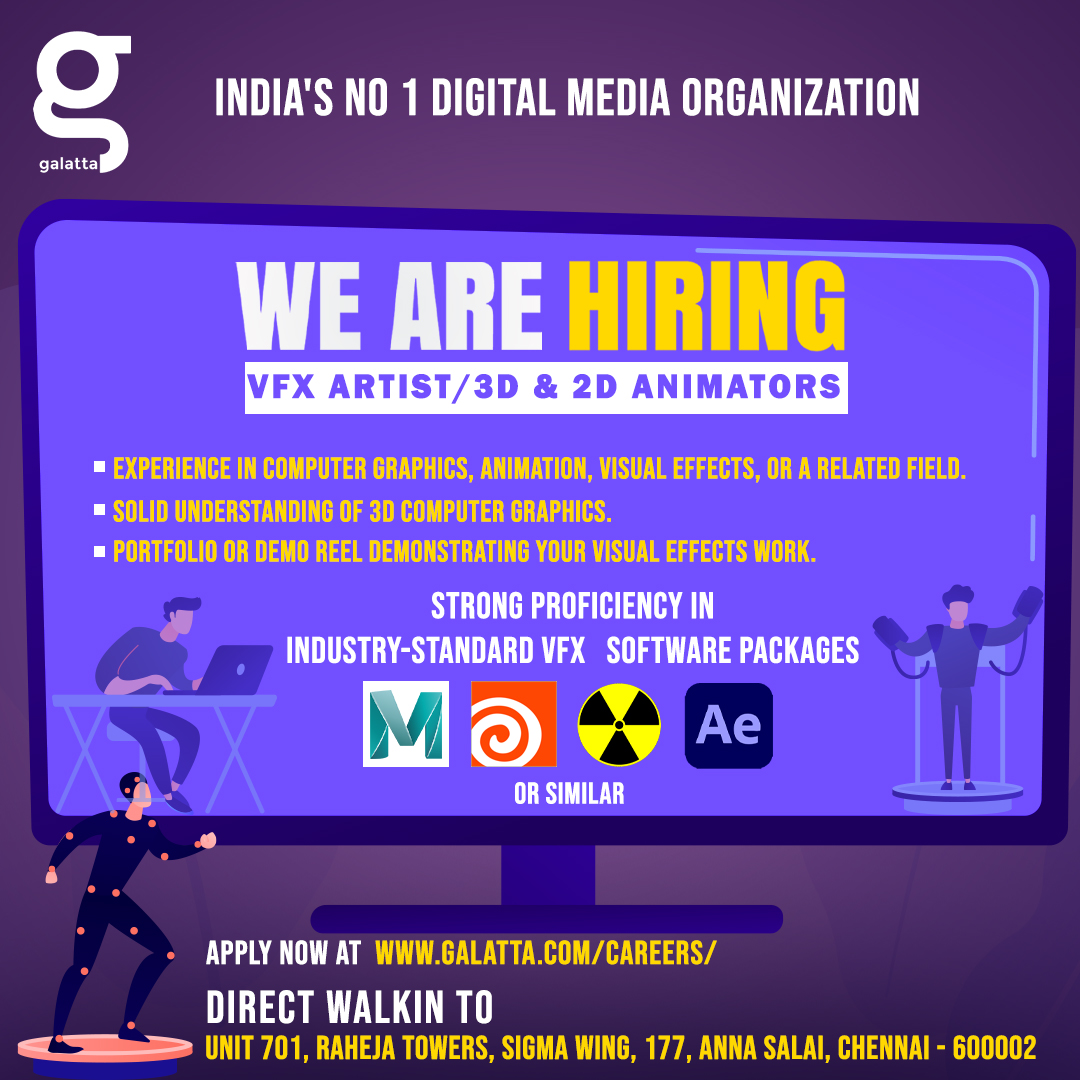The image is a scan of a digital advertisement against a dark purple background. In the top left corner, a logo featuring a lowercase 'g' followed by the lowercase word "Galata" is prominently displayed. To the right of the logo, in white text, it reads: "India's number one digital media organization." Below this header, a minimalist cartoon drawing of a computer monitor, with a brighter purple screen, contains the recruitment announcement. In white text, it says: "We are hiring," with "hiring" emphasized in bright yellow. Additionally, "VFX artists / 3D and 2D animators" is written inside a white box in purple text. Further down, the advertisement details the job requirements in yellow text: "Experience in computer graphics, animation, visual effects, or a related field. Solid understanding of 3D computer graphics. Portfolio or demo reel demonstrating your visual effects work." Beneath these texts, it continues in white: "Strong proficiency in industry-standard VFX software packages." The bottom of the advert features additional details along with graphical representations of people working at computers, using VR software, and engaging in motion capture.